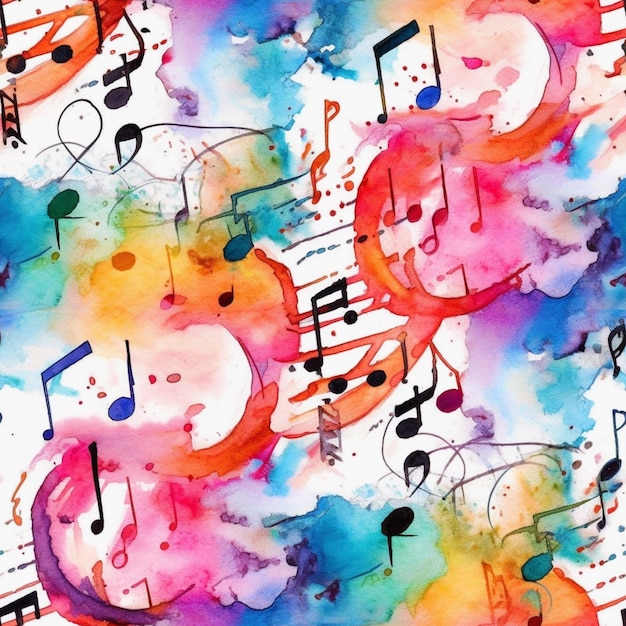This image is an abstract, cartoonish watercolor painting, brimming with a kaleidoscope of colors and musical notes that seem to float in the air. The upper left-hand corner features orange swirls interspersed with black musical notes, ranging from sixteenth notes with double flags to quarter notes without any flags. Moving towards the middle, the painting transitions into hues of purple, blue, and green, mingling seamlessly with more orange and darker red. A variety of musical notes—black, brown, and blue—are scattered throughout, some aligned with colorful lines that resemble musical staves. The bottom of the painting showcases an array of colors: yellows on one side, blues in the center, and pinks to the left, each accompanied by more floating musical notes. The backdrop is predominantly white, allowing the vibrant watercolors to blend and transition into each other, creating an impression of music and color suspended in the air.